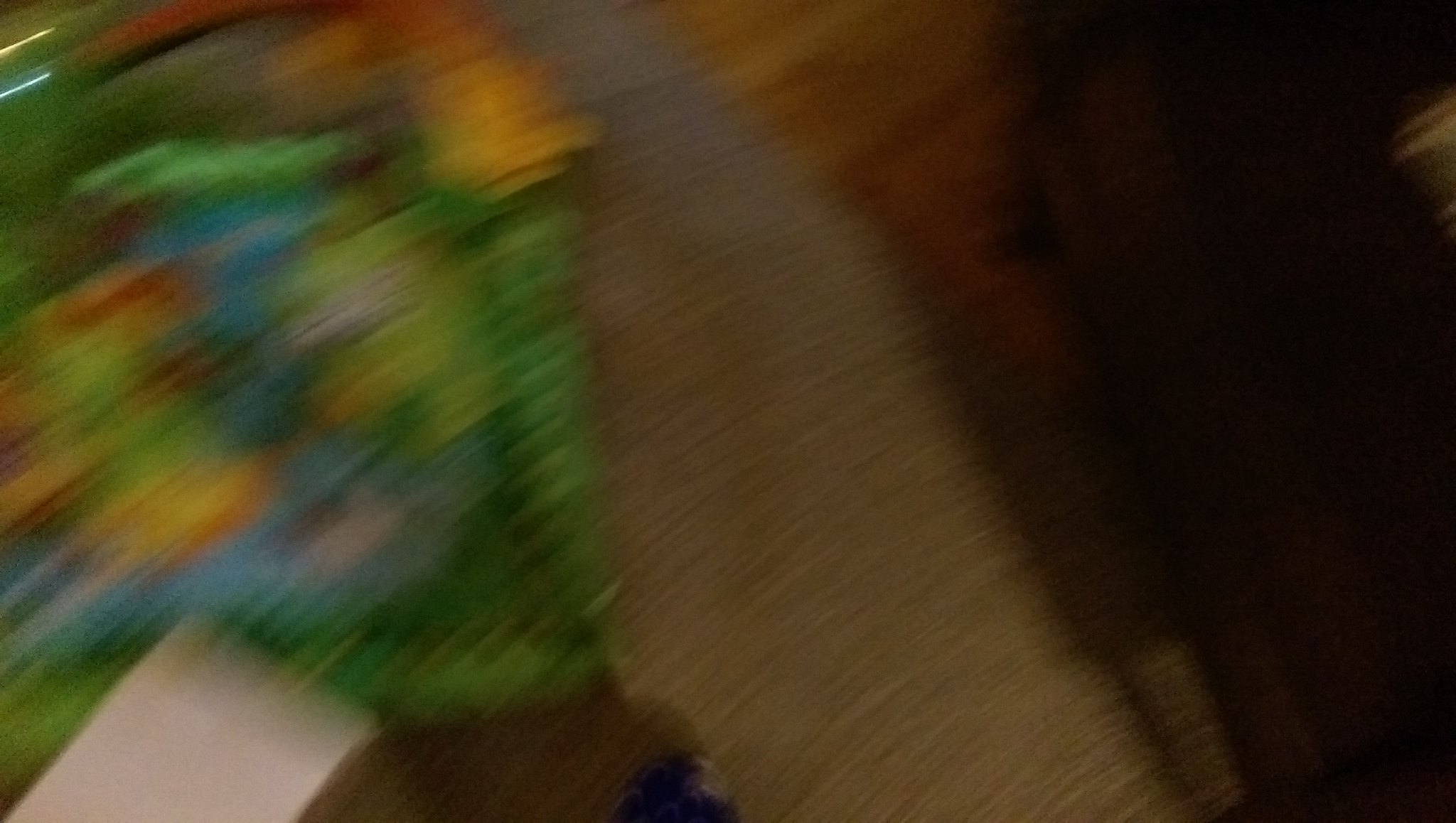The image appears to be a slightly blurred scene composed of various elements. On the left side, there are vibrant patches of green, blue, yellow, and red, suggesting some colorful, possibly out-of-focus objects or decorations. Intermixed with these colors is a piece of white paper, contrasting against the vibrant hues. There's also an area illuminated by light at the top of the image, adding a diffuse glow. Moving to the right, the image transitions to a darker tone with a section of black asphalt, likely a road or path, accompanied by scattered black shadows, which could be cast by nearby objects or people. Interspersed between these elements is a piece of wood, adding a natural texture to the scene. The overall composition suggests an outdoor setting with a mix of natural and man-made elements, captured in a moment of motion or with a focus on abstract details rather than clear, distinct forms.